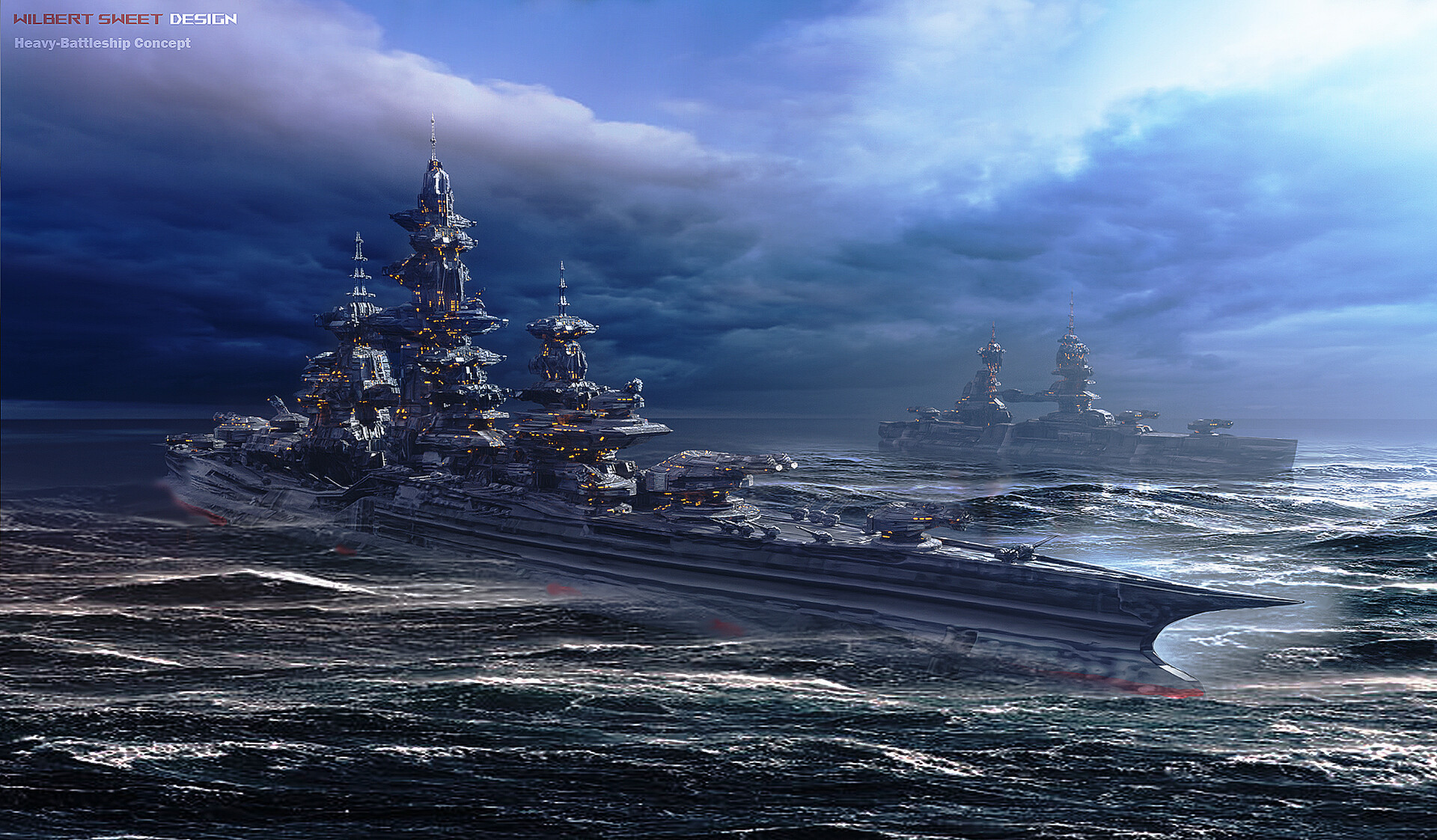The image is a highly realistic depiction or rendering of a technologically advanced, fictional heavy battleship concept known as the "Hilbert Sheet Design." The artwork, marked by dark, turbulent ocean waves and a stormy sky thick with clouds, showcases two massive battleships slicing through the sea. Towering structures rise from each ship, resembling alien skyscrapers with rounded forms, giving the appearance of entire cities floating in the ocean. The scene is predominantly dark, punctuated only by subtle sunlight and rain. Both ships, long and metal with sharp bows, exude an otherworldy, almost alien design that distinguishes them from any known real-life vessels. Text featured in the top left corner of the image includes "Hilbert Sheet Design" in red lettering, "Design" in white, and "Heavy Battleship Concept" in transparent text, solidifying its conceptual and imaginative nature.